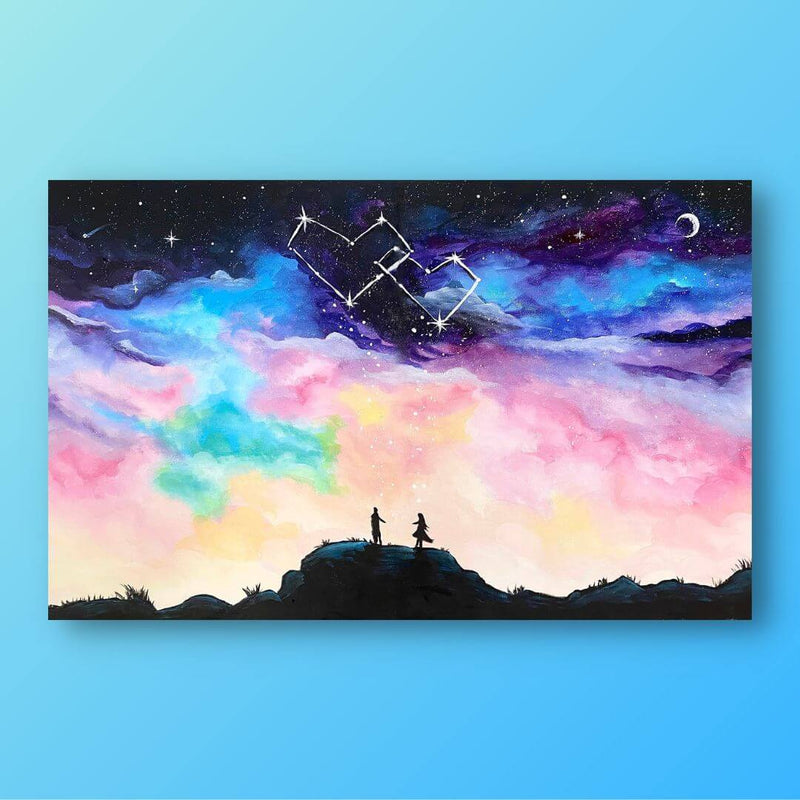The painting is mounted on a vibrant neon blue wall and depicts a striking landscape, presented in a horizontal, rectangular format. Dominating the lower part of the painting is a black silhouette of a cliffside hill with a prominent rock at its center. Standing on the rock are two tiny, stick-figure silhouettes—a man and a woman, seemingly on the verge of an embrace. The woman, dressed in a full skirt, appears to be spinning, while the man extends a hand towards her.

The sky behind them is a cascade of vivid colors, transitioning from a vibrant pink with hints of yellow at the horizon to a deep and rich purple. Higher up, the sky darkens to a deep blue and finally to black, speckled with numerous white stars, including a noticeable shooting star and a crescent moon in the upper right corner. At the center of the sky, two overlapping hearts are depicted, formed by white lines connecting star shapes, with a larger heart enveloping a smaller one on the right.

The background of the overall painting is a calming teal-blue, suggesting that it might be hand-painted on canvas with watercolor. The celestial elements and the interlinked hearts add a sense of whimsy and romance to the ethereal scene, making it a captivating piece of art that blends simplicity with striking, vivid details.